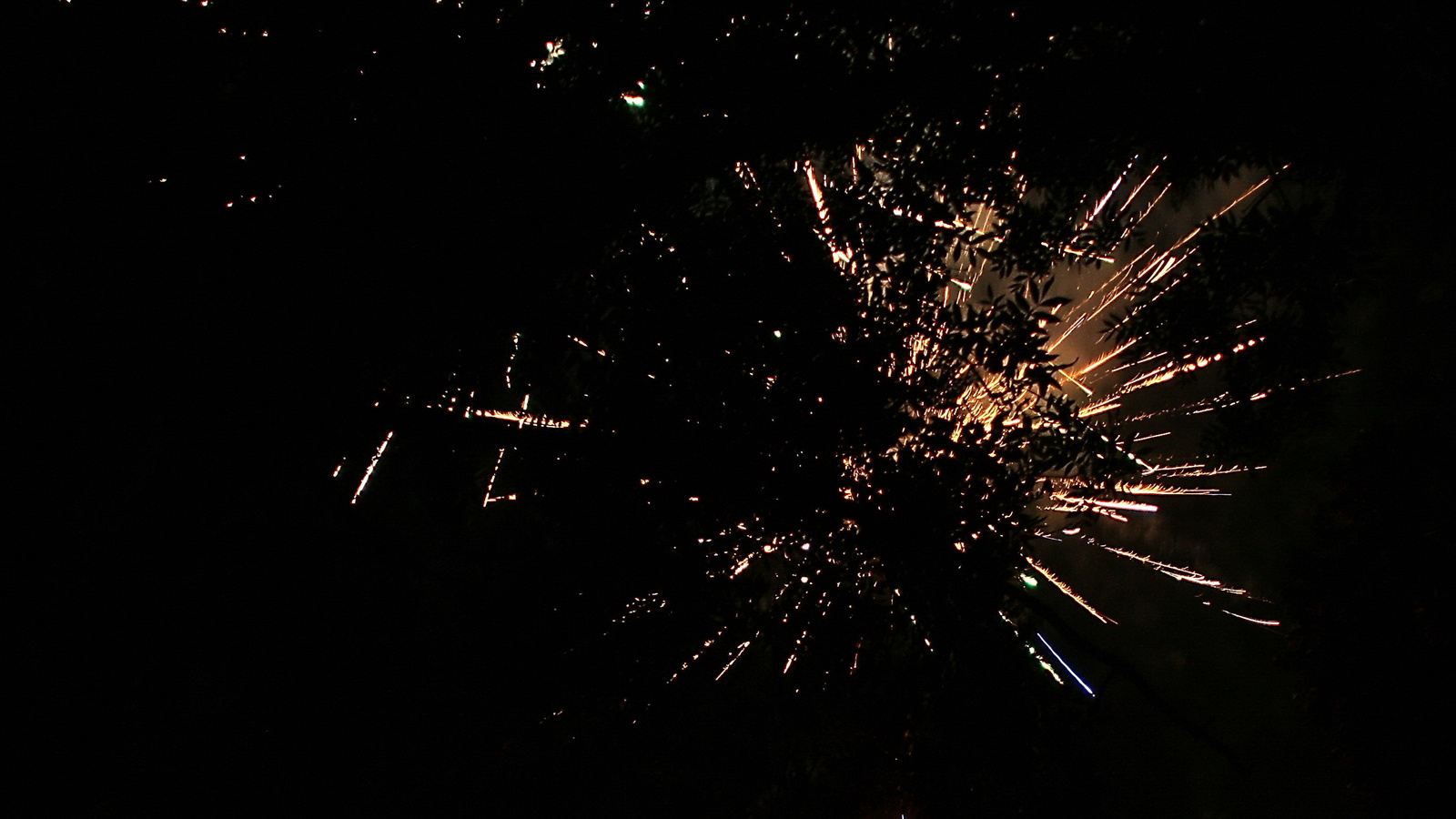The image depicts an abstract scene dominated by a black background interspersed with splashes of brown, gold, white, green, yellow, and gray. The overall impression gives the sense of dynamic, impressionistic bursts of color across a dark canvas. In the middle-right section of the picture, there are faint, shadowy shapes resembling fern leaves or tree foliage, which seem to emerge from the darkest part of the image. This interplay of light and shadow creates the illusion of leaves casting shadows. The streaks and specks of light are scattered chaotically, evoking the appearance of an exploding meteor or asteroid, or even a scene of welding sparks flying. Despite its seemingly chaotic nature, the image lacks a definitive object or focal point, leaving its interpretation entirely open to the viewer.